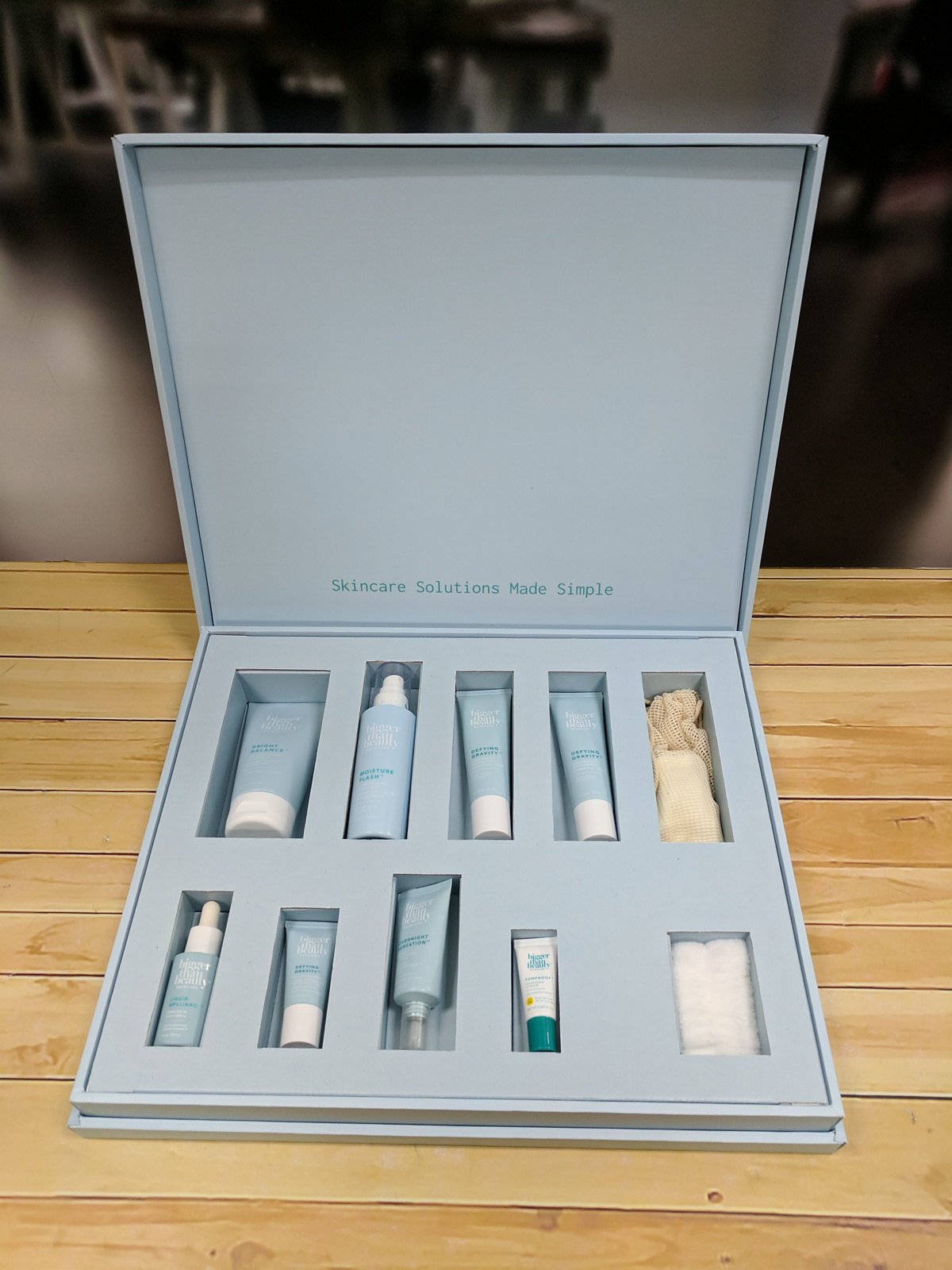The image features a slim, square, light blue box with a lid that lifts open to reveal ten compartments, each containing a beauty product. The products appear to be uniformly light blue in color. The box, labeled with the words "Skin Care Solutions Made Simple" (though the text is small and somewhat difficult to read), houses a variety of skincare items. Notably, there are three small tubes that may contain foundation or another type of skincare cream. The box is positioned on a light-colored wooden table, with blurred objects faintly visible in the background. This organized and aesthetically pleasing kit offers an array of skincare solutions, all neatly presented in a chic blue container.